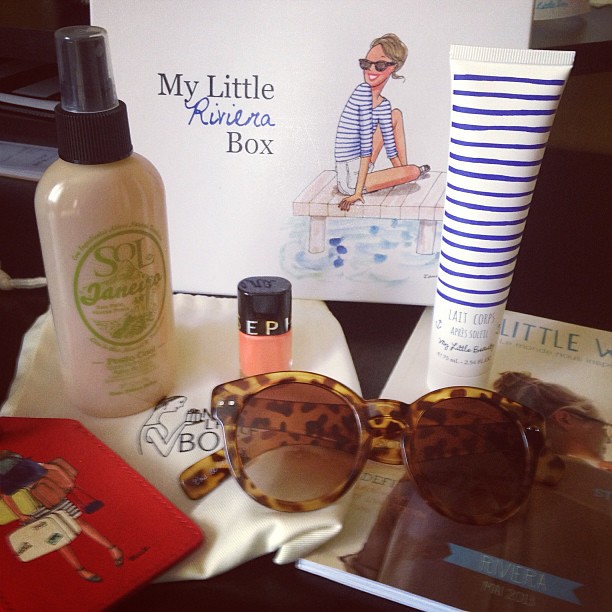On the countertop, an array of beauty and travel-themed items are meticulously arranged. Starting from the left, there's a red luggage tag featuring an illustration of a girl burdened with multiple suitcases. Adjacent to it lies a white travel bag, atop which rests a distinctive beauty spray bottle labeled "Sol Janeiro" in translucent packaging with green text. Nearby, there's a bottle of pink nail polish. Centrally positioned in the photo is a pair of leopard-patterned sunglasses. Flanking the items on the right are a tall white tube with blue stripes inscribed "Lait Corps" and a small magazine. In the backdrop, the display is crowned by a lid that reads "My Little Riviera Box," adorned with a drawing of a woman donning sunglasses, relaxing on a wooden dock by the water.